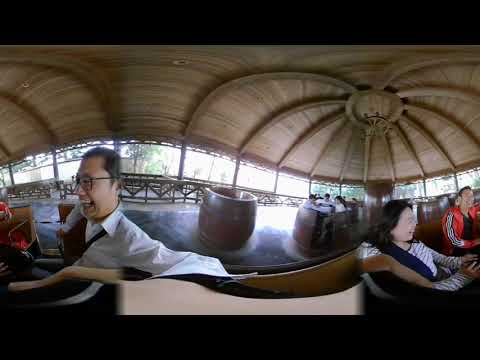The horizontally aligned panoramic image captures a lively scene at an amusement park, where people are enjoying a spinning cup ride under a complex wooden domed ceiling. The ride is designed with several circular booths along the edges, where participants sit, creating a barrel-like appearance. The picture prominently features a cup in the foreground, occupied by three individuals all laughing and smiling. On the left side, a man wearing a white button-down dress shirt and glasses rests his arms on the edge of the cup, clearly amused. To the right, a woman with shoulder-length black hair, wearing glasses and a striped long-sleeve shirt, laughs heartily. Next to her, another man with short, dark hair sports a red jacket with white stripes down the sleeves, also caught in the joy of the moment. In the background, the open areas between the domed sections reveal a glimpse of trees and bright sky, adding a natural contrast to the amusement park's festive atmosphere.